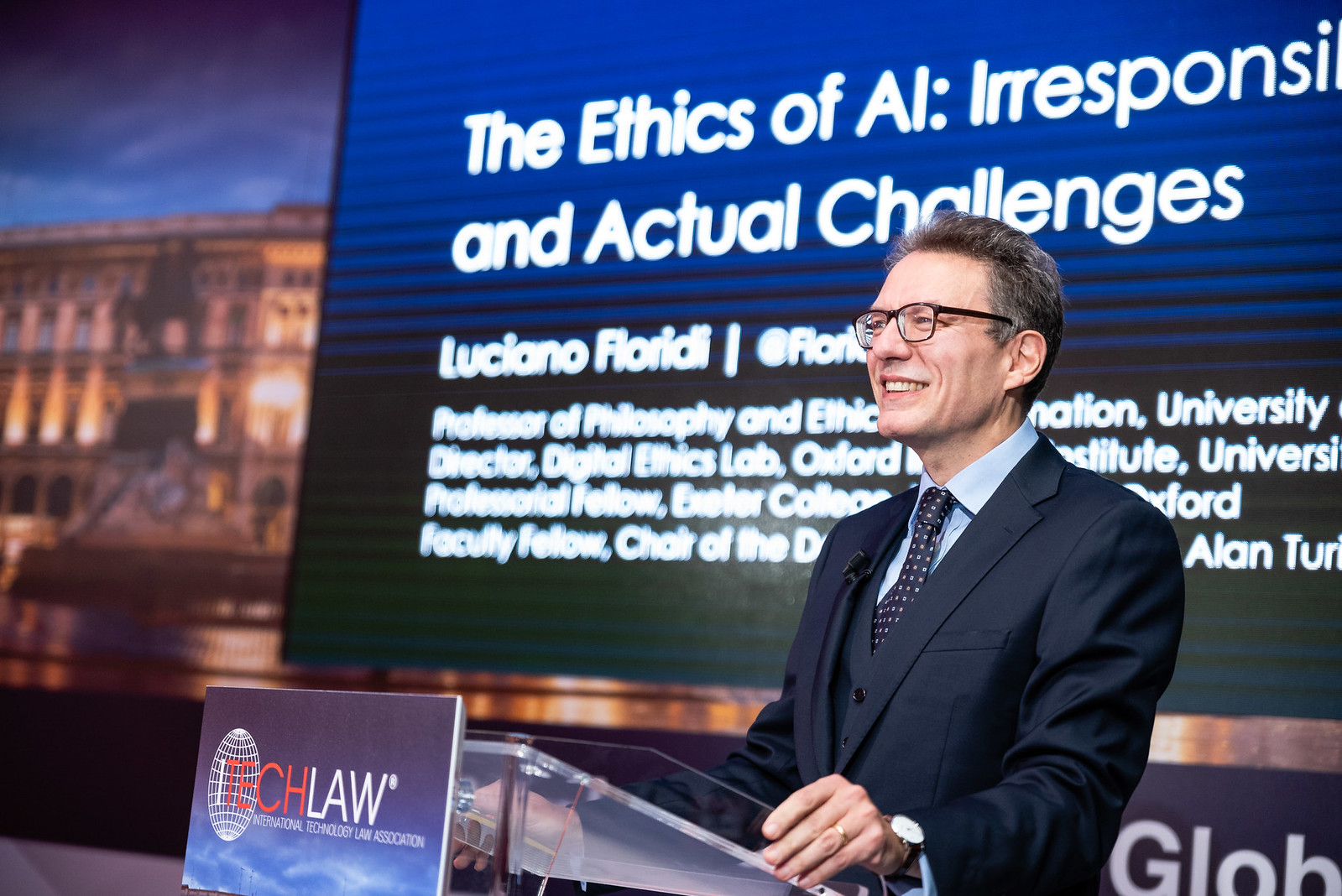In this detailed image, a distinguished man is presenting at a conference behind a podium labeled with "Tech Law," where "Tech" is in red and "Law" in white, accompanied by a globe-like symbol. The speaker, identified as Luciano Floridi, is a Caucasian gentleman dressed professionally in a dark blue suit, light blue shirt, and a purple polka-dotted tie. He also wears glasses and sports a good-natured smile, giving him a professorial appearance. The backdrop features a slanted modern blue billboard with white text that reads: "The Ethics of AI: Irresponsible and Actual Challenges." His name and titles, partially obscured by his body, denote him as the Professor of Philosophy and Ethics and Director of Digital Ethics Lab at Oxford, among other affiliations. The upper left background seems to depict a large, illuminated building with a statue, though it's slightly blurred. The overall scene is rich with vivid blues, blacks, and whites, reflecting a sophisticated, modern aesthetic suitable for a professional setting.